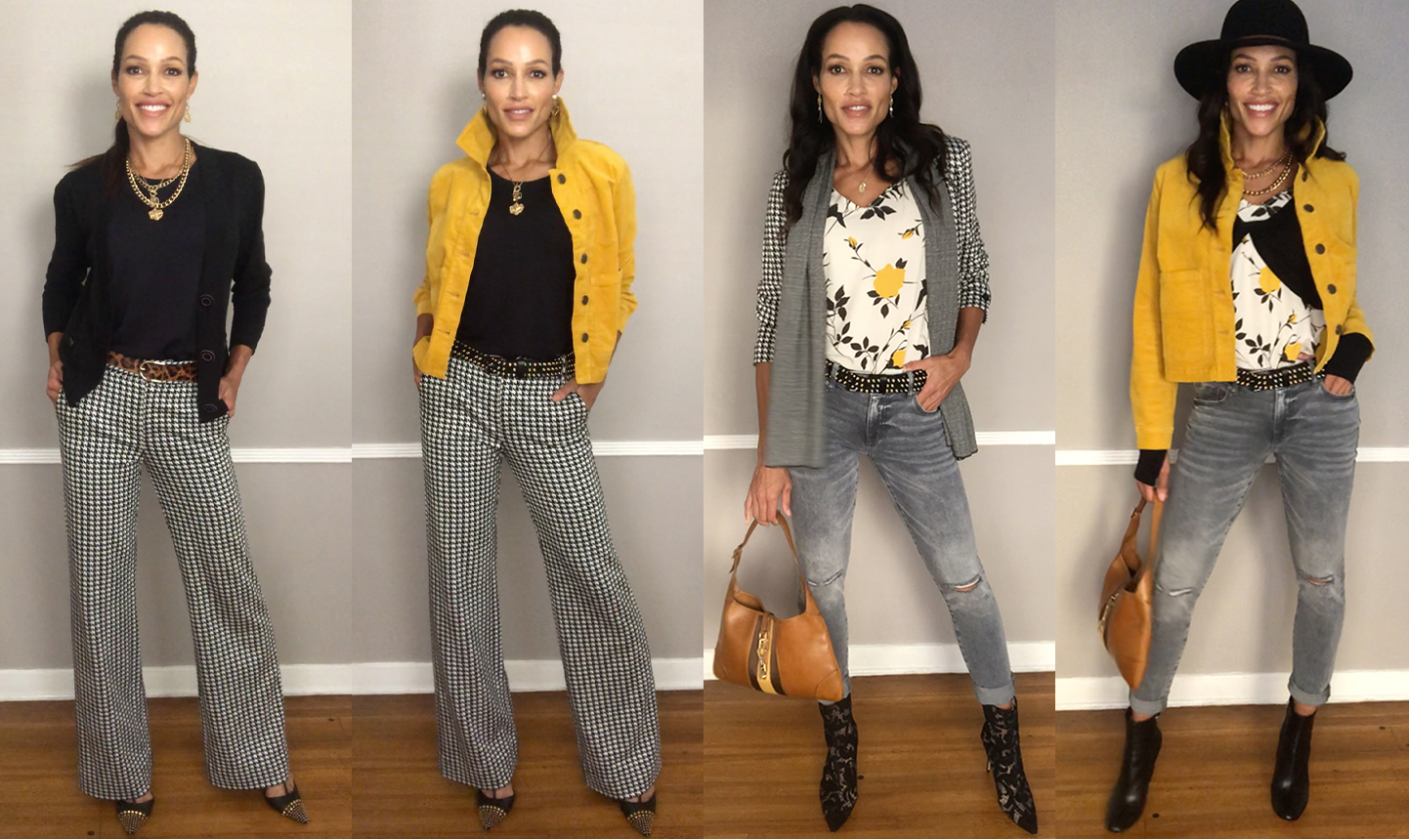The image is a compilation of four photographs featuring a tall, dark-skinned model with a radiant smile, captured in a stylish indoor setting with a wooden floor and a gray backdrop. In each image, she showcases variations on a chic, mix-and-match wardrobe. Her hair is pulled back in the first two images, where she dons a sleek black shirt paired with black and white checkered pants. In the first picture, she accentuates her look with a black blazer and a leopard print belt. In the second, she adds a pop of color with a bright yellow jacket and a black checkered belt.

In the third and fourth photographs, her style evolves with a switch to grayish jeans featuring ripped knees, and classic black boots. She sports a white t-shirt adorned with a yellow fruit design, layered under different outerwear. The third image highlights a gray scarf and a pocketbook, while the fourth repeats the bright yellow jacket from the second image, adding a cerulean leather bag and a black hat for a playful twist. Throughout all the images, her confident stance with hands in her pockets and her joyful expression, enhanced by makeup and gold jewelry, suggest a vibrant lesson in fashion versatility.